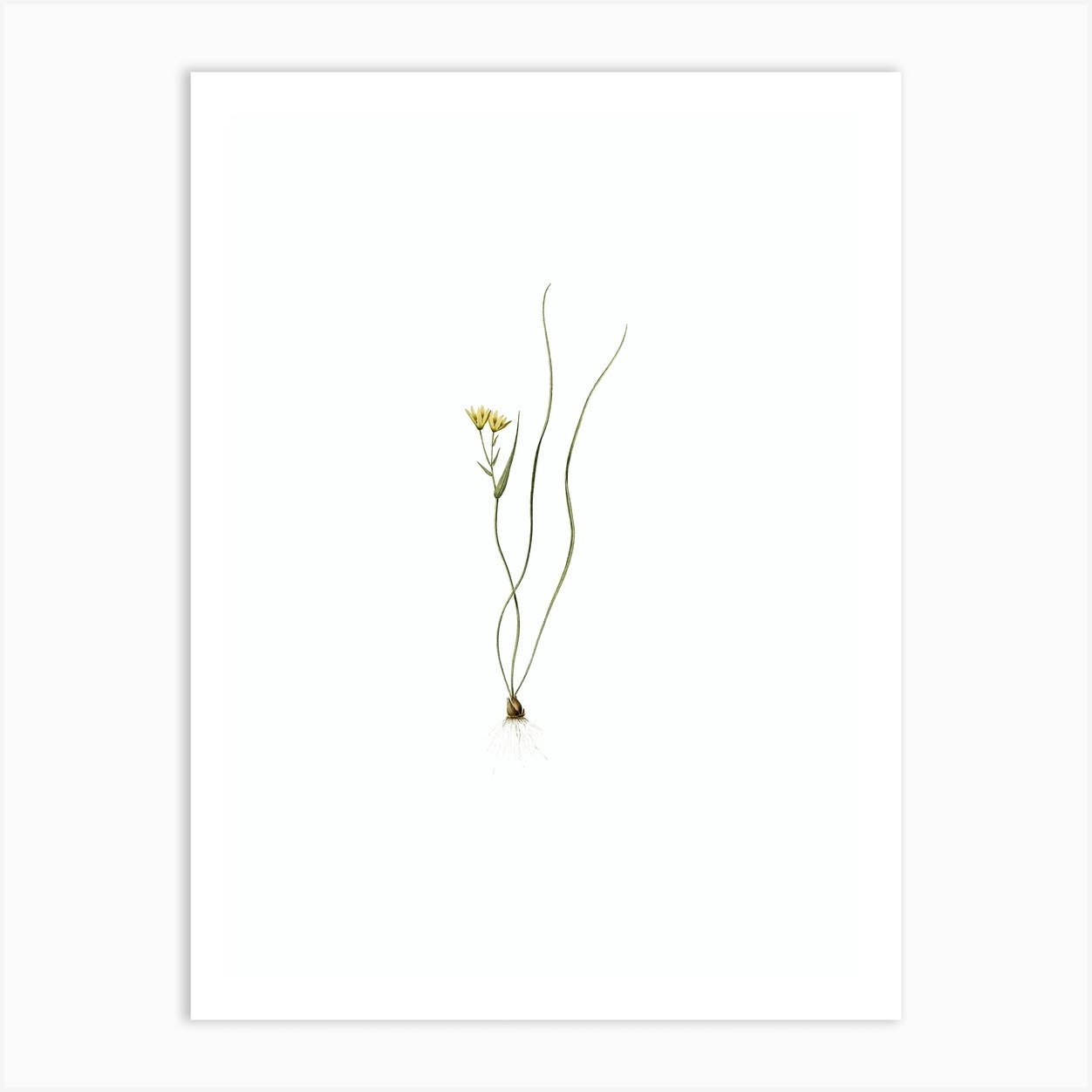This is a simple yet detailed digital drawing set against a solid white background. The central focus is a delicate plant growing from a bulb with visible, faint roots at the bottom. Three slender stems rise from the bulb, with two curving gracefully to the right and one to the left. The rightward stems are bare and slightly wavy, while the leftward stem supports a long, thin leaf and two animated, upward-facing yellow flowers with darker centers. The arrangement of the stems slightly resembles the back legs of a woman, adding a subtle artistic touch. The overall composition is tranquil and quiet, devoid of any text or human figures.